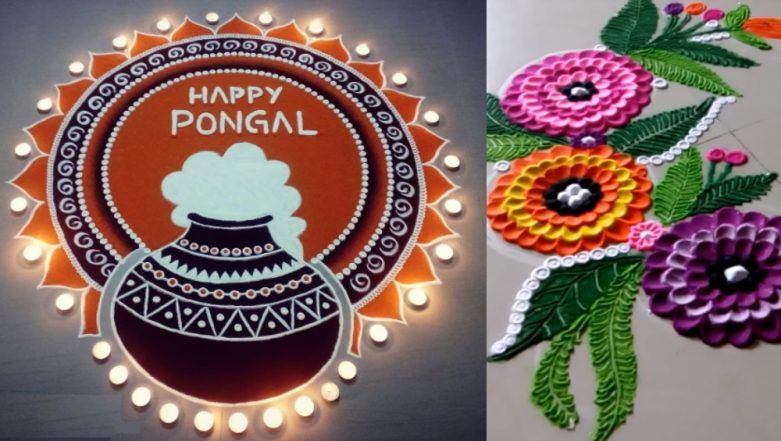The image consists of two adjacent photographs. The left photograph features an ethnic, Indian-themed artwork with a large orange circle surrounded by a brown border, decorated like a sunflower with brown petals extending outward. At the base of the circle, there's a brown vase emitting a white, fluffy substance, with "Happy Pongal" inscribed in white text at the center. The artwork is adorned with light bulbs or candles around the edges, adding to the festive feel, and incorporates additional intricate patterns including dots, swirls, and triangles in a color scheme of black, white, orange, and red.

The right photograph displays a gray floor embellished with a fabric carpet or a decorative piece of flowers. The arrangement includes a variety of vibrant flowers: one large one—orange and yellow with a black and white center—and multiple smaller ones in shades of purple, dark purple, light pink, and dark pink, each with detailed central elements. Among these, there are also green leaves sprouting in various directions, enhancing the lively, dynamic composition. These fabric flowers are arranged three-dimensionally, providing a rich texture against the flat, gray surface.